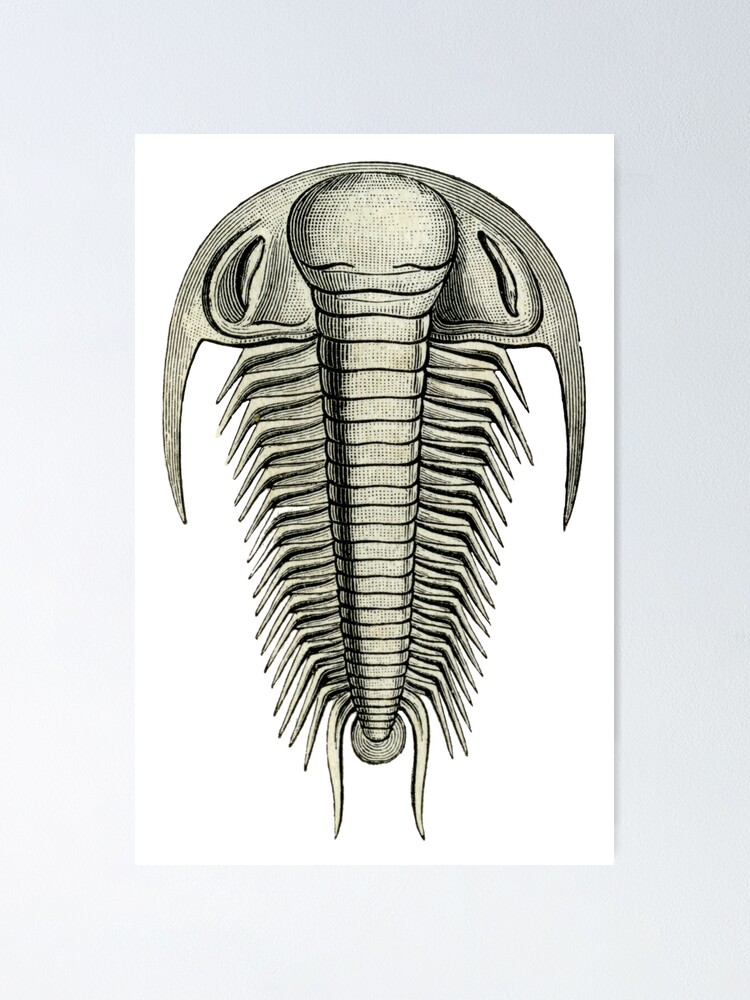This image showcases a detailed illustration of a fossilized trilobite, rendered in a Pointillism ink technique that employs shades of pale taupe and light gray. The trilobite's body features a prominent, tapering spine running down the center, flanked by numerous, small pointy appendages arranged in many rows that bend downward at the middle point, resembling a series of bones or a rib cage. Its head is oval-shaped, forming a half-moon that terminates in downward-pointing mandibles on each end. The creature's lateral sides bristle with dozens of delicate legs extending from the central segmented body. Black ink highlights and subtle darker shades are used to delineate the different parts, adding to the texture and depth of the portrayal. The illustration, set against a white background, is placed on a white surface, bordered by a light gray backdrop, enhancing the contrast and intricacy of the sketch.